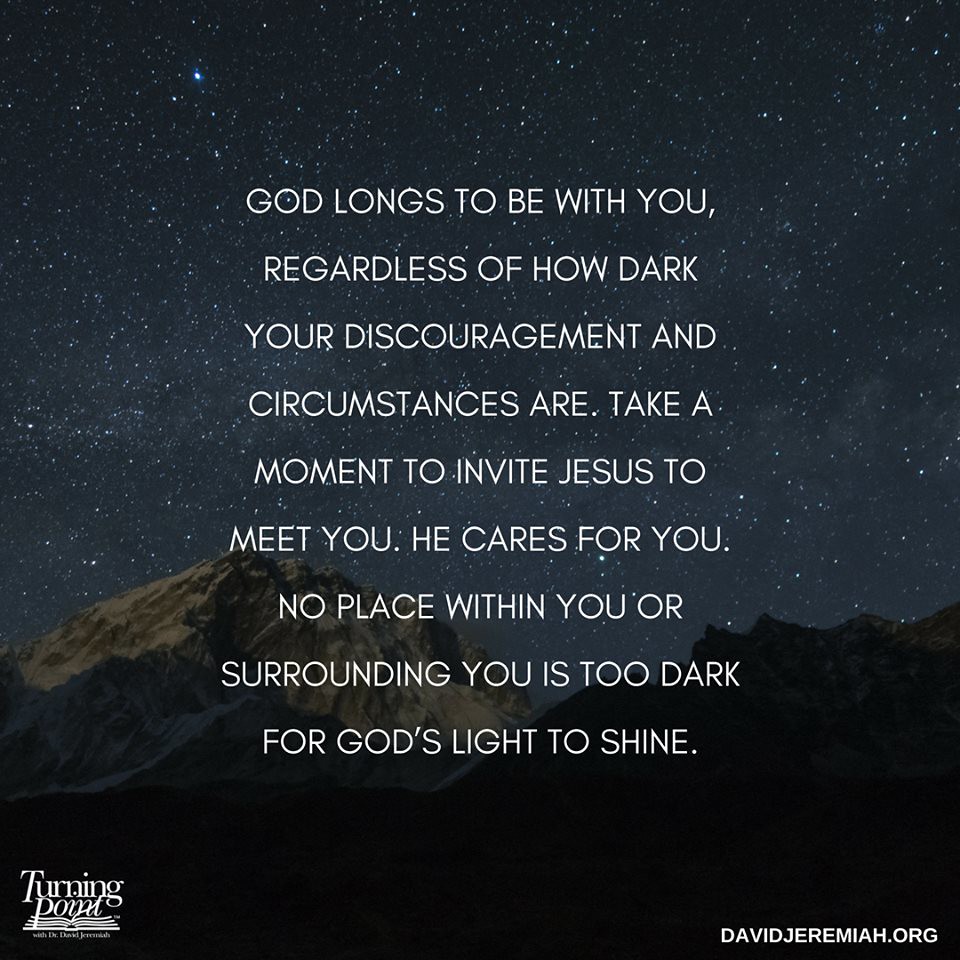The square image features a nighttime sky with a charcoal hue, sprinkled with tiny white specks resembling stars, creating a serene celestial backdrop over a silhouette of mountains. Centered in the image are eight to nine lines of text in all-capital white letters, boldly stating: "God longs to be with you regardless of how dark your discouragement and circumstances are. Take a moment to invite Jesus to meet you. He cares for you. No place within you or surrounding you is too dark for God's light to shine." At the bottom left-hand corner, there's a logo for Turning Point, featuring an image of an open book beneath the text. In the lower right-hand corner, "DAVIDJEREMIAH.ORG" is prominently displayed in white, all-capital letters, indicating the website's origin. The overall aesthetic and messaging are designed for religious encouragement, suitable for social media sharing among Christian audiences.